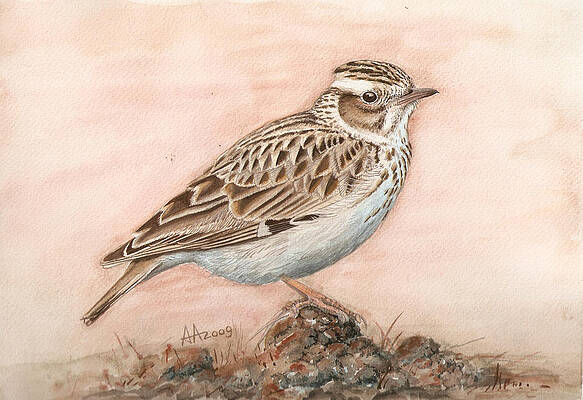The illustration depicts a small bird resembling a sparrow, perched on a small pile of stones and earth. This bird is shown in a profile shot, with a white belly, brown plumage, and various shades of brown and white on its head, face, neck, feathers, and tail. It has distinctive brown and white striped patterns on the top of its head, a black beady eye, and a pointed narrow beak. The bird's orange feet are propped up on the stones, which are colored in shades of gray, brown, and red, with small lines likely representing grass or weeds. The background of the drawing is a mottled peach and white color, creating a neutral tan tone. Below the bird, just above the rocky terrain, there is text that reads "AA2009" in a light brown shade. A possible signature is also visible in the lower right-hand corner, though it is not easily readable.